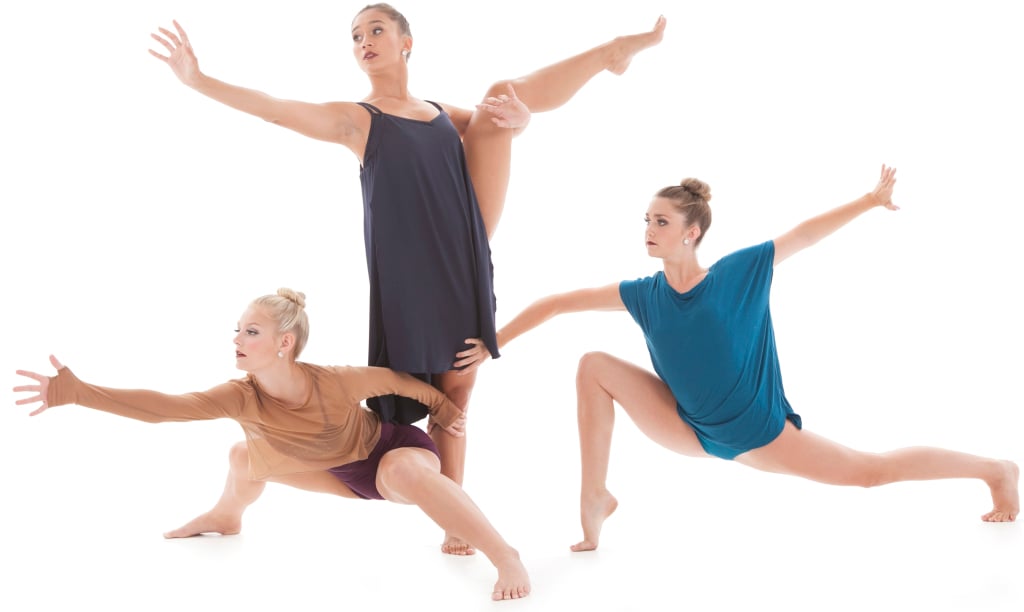The image showcases three women performing yoga-like dance poses against a complete white background. All three have their hair styled in high buns and wear dark red lipstick, white earrings, and dramatic eye makeup with dark eyeliner and mascara. The woman on the left, a blonde in a tan long-sleeved shirt and purple shorts, is in a deep sumo squat with her legs spread wide apart. Her right hand is extended forward toward the left side of the image, and her left hand is placed on the leg of the middle woman. The middle dancer stands on her right leg while holding her raised left leg with her left hand. She is dressed in a flowy, dark purple spaghetti strap dress and is looking and reaching out to the left with her right arm extended. The woman on the right, wearing a flowy, bluish-teal top that resembles a one-piece dress, is in an extended lunge position with both hands extended outward. Her right hand supports the leg of the middle dancer while her left arm reaches behind her towards her bent back leg. Each of the women embodies a unique pose, yet they are interconnected through their movements and touches.